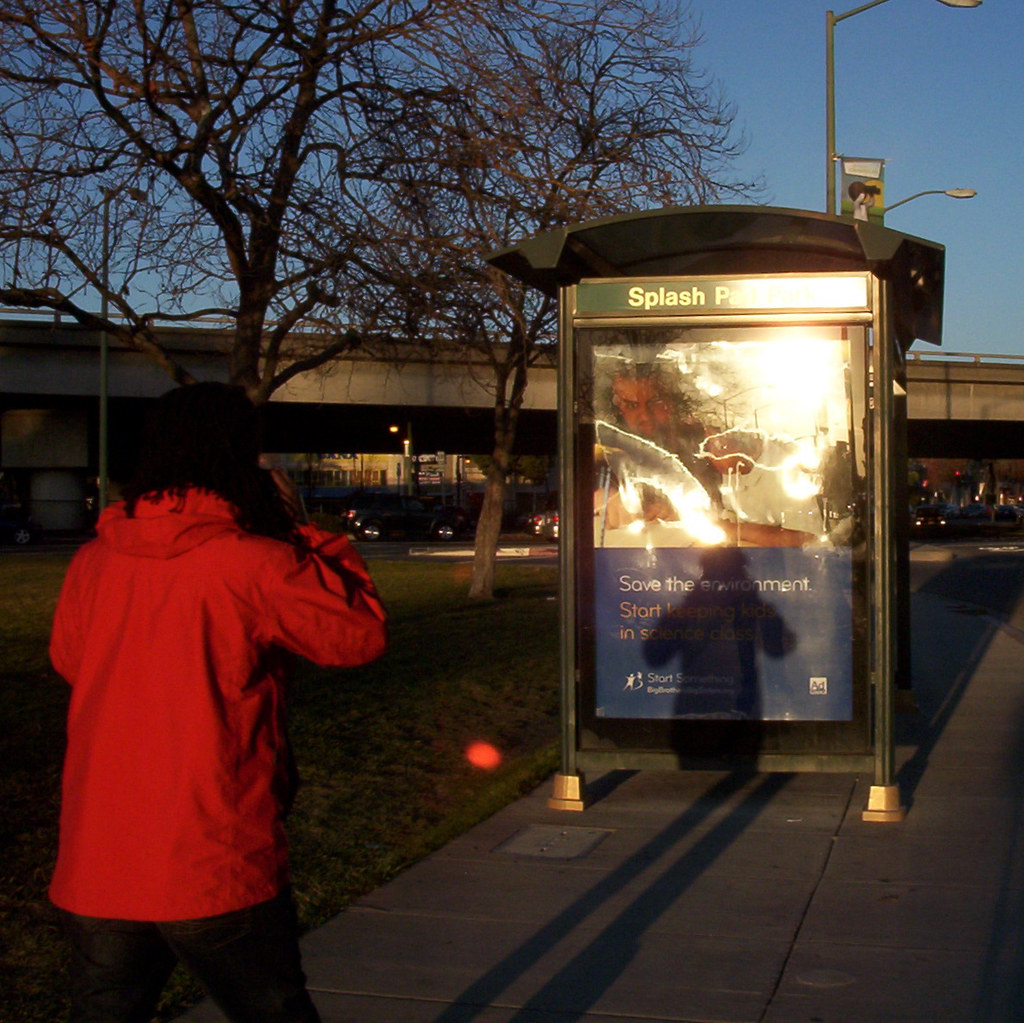This photograph captures a serene urban scene, likely taken during the early morning or late evening given the soft lighting and slight glare from the sun, indicating it is either rising or setting. Central to the image is a street upon which an individual is walking away from the viewer. The individual is dressed in a bright red jacket, dark jeans, and possibly a black hat. To the left of the street, there is a green metal bus stop with an encased glass advertisement that reads "SPLASH PAD PARK," but glare makes further details hard to discern. Adjacent to the bus stop is a grassy ground dotted with trees. Beyond this area, in the distance, there is a road bustling with several vehicles, and above it arches a highway bridge. The scene is bathed in the soft tones of a clear, blue sky, and illuminated by a streetlight, adding to the tranquil yet dynamic urban landscape.